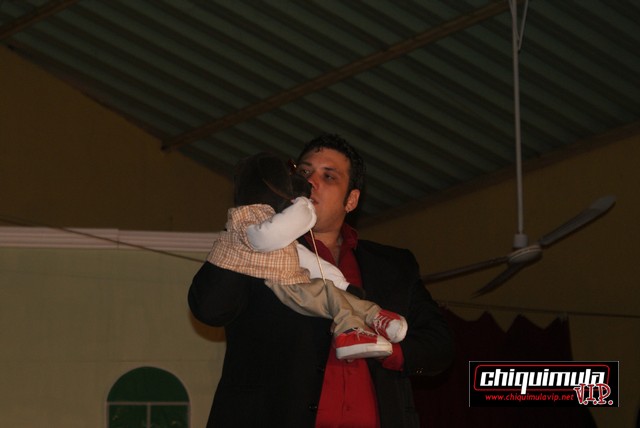In the image, a man in his 30s with black hair is wearing a black suit jacket over a red button-down shirt. He is holding a puppet that resembles a small child or a puppy dog, dressed in an orange and white striped coat, khaki pants, and red sneakers. The man is engaging with the puppet, holding its face close to his as if in conversation, suggesting he may be a ventriloquist performing a comedic routine. They are situated in what appears to be the interior of a building, visible through its green roof with brown diagonal beams. A white ceiling fan with three blades is suspended from the ceiling. In the image's lower right corner, "CHIQUIMULA VIP" is written in white and red text, alongside a website URL.